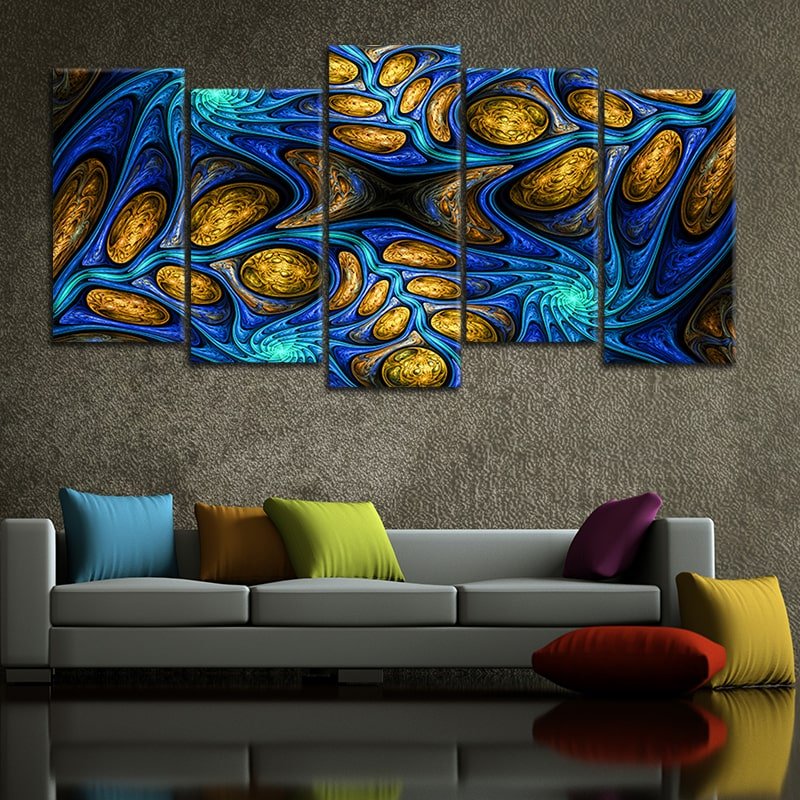This image presents a modern, possibly computer-generated, living room scene featuring a gray sofa situated against a textured gray wall, which has a carpet-like appearance. The wall hosts five tall, rectangular paintings, each positioned closely and forming a cohesive, abstract artwork. This artwork showcases a stunning composition of gold and yellow ovals interspersed with vibrant blue and green hues, depicting shapes reminiscent of dragon wings or cellular structures. The glossy, almost mirror-like black floor reflects the gray couch, enhancing the room's modern aesthetic. The couch itself is adorned with four scattered pillows in varying colors: blue, golden-orange, lime-green, and purple. Additionally, two more pillows—a red and a gold one—are casually placed on the floor in front of the sofa. The overall decor blends bright, vibrant elements with a sleek, contemporary setting, creating a striking visual impact.